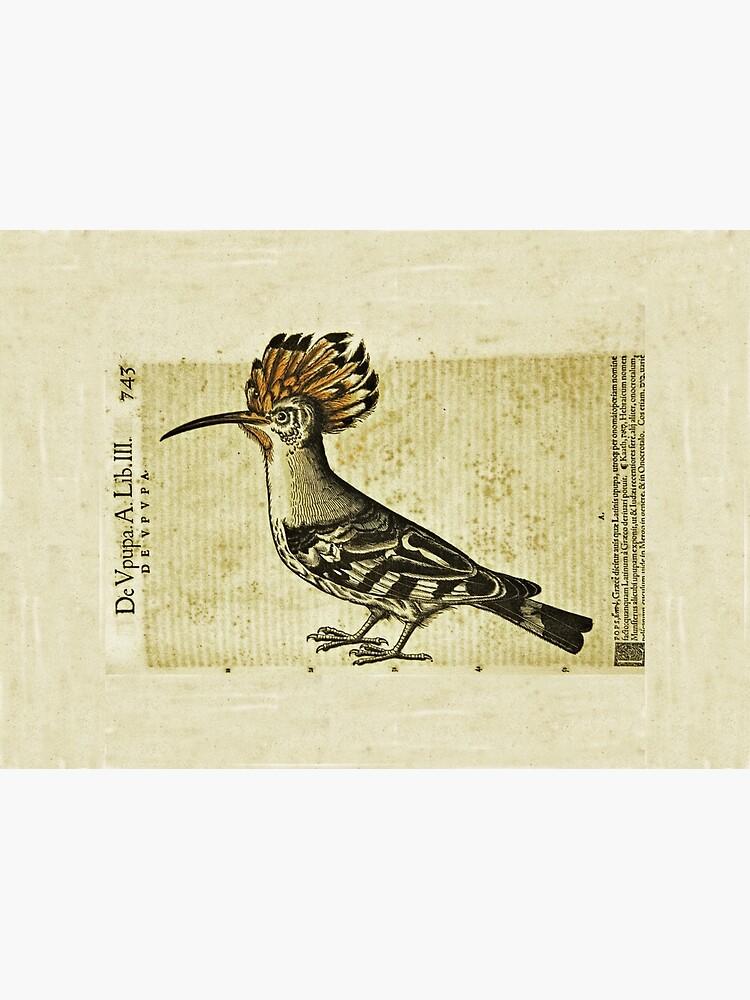This image presents an artistic depiction of a bird, positioned prominently at the center of a tea-stained beige rectangular background, reminiscent of an aged postcard or a novel page. The bird, illustrated in vibrant detail, features a strikingly long and curved beak, black with an orange base near its face. The bird's head is adorned with an elaborate crest of orange feathers tipped in black, giving it a regal appearance. The eyes are keen and attentive, enhancing its vivid charm.

The bird's plumage includes a white throat transitioning to black as it extends around the neck, with the chest displaying a mix of white and black lines. The wings are adorned with bold black and white stripes, adding to the bird's striking visual contrast. The tail features predominantly black feathers with hints of other colors, adding length and balance to its form.

Two talons are visible, grounding the bird realistically on the tan paper. To the left of the bird, there is a block of text that reads "D.E.V.P.U.P.A. A.L.I.B III" along with the number "743," all tilted slightly to the left. Additional smaller text in an untranslated language is also present, enhancing the vintage and mysterious allure of the piece. The overall composition blends detailed artistry with a hint of scholarly antiquity, making the illustration both visually captivating and texturally rich.